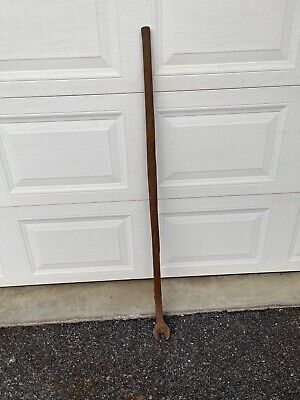The image showcases a close-up view of a typical white garage door adorned with textured, engraved rectangular panels. In front of the door lies a black asphalt driveway that meets a small cement apron at the garage's base. Leaning against the garage door is a long, rusted brown metal tool with a curved, wrench-like end, possibly meant for unscrewing or reaching fasteners. The handle of this tool rests on the driveway, emphasizing its considerable length. This simple, unembellished scene focuses solely on the garage door and the unusual tool, suggesting an everyday residential setting.